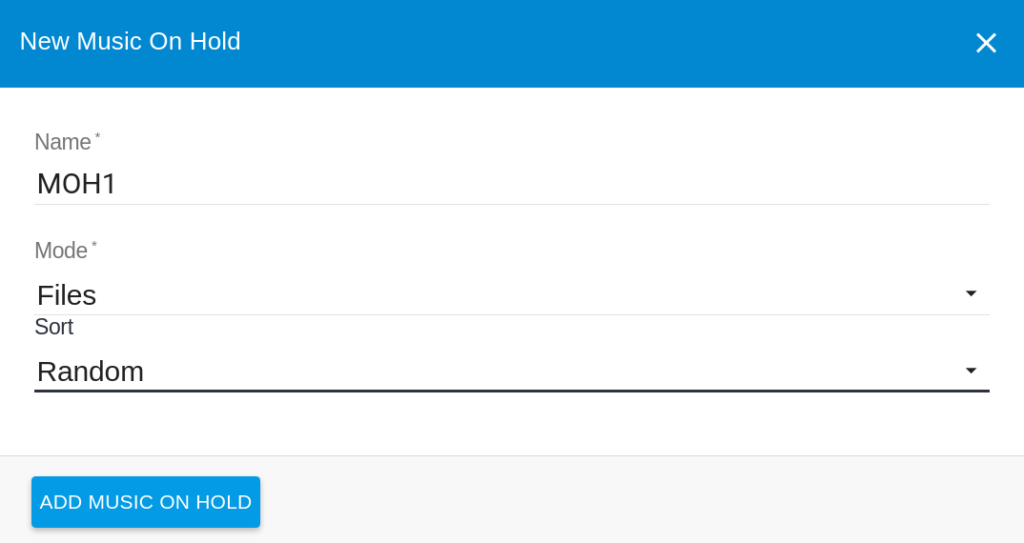The image depicts a music management web page, possibly related to a music-on-hold system. At the top, a large blue horizontal banner spans the entire width of the page. On the right side of this banner is a white "X," while on the left, white text announces "New Music on Hold."

Below this header, there is a form section with several interactive elements. The first field is labeled "Name," where the text "MOH1" has been entered. Beneath this, another field labeled "Mode" shows a downward-pointing arrow, indicating a dropdown menu, with "Files" selected. Following this, a "Sort" field—also accompanied by a downward-pointing arrow for a dropdown menu—has "Random" chosen.

At the bottom of the page, within a smaller blue button located in the lower-left corner of a larger white rectangle, the text "Add Music on Hold" is displayed in white. This clickable button appears to be a call to action to finalize or add the specified settings.

The overall layout is clean and straightforward, designed to facilitate easy management of music-on-hold configurations.